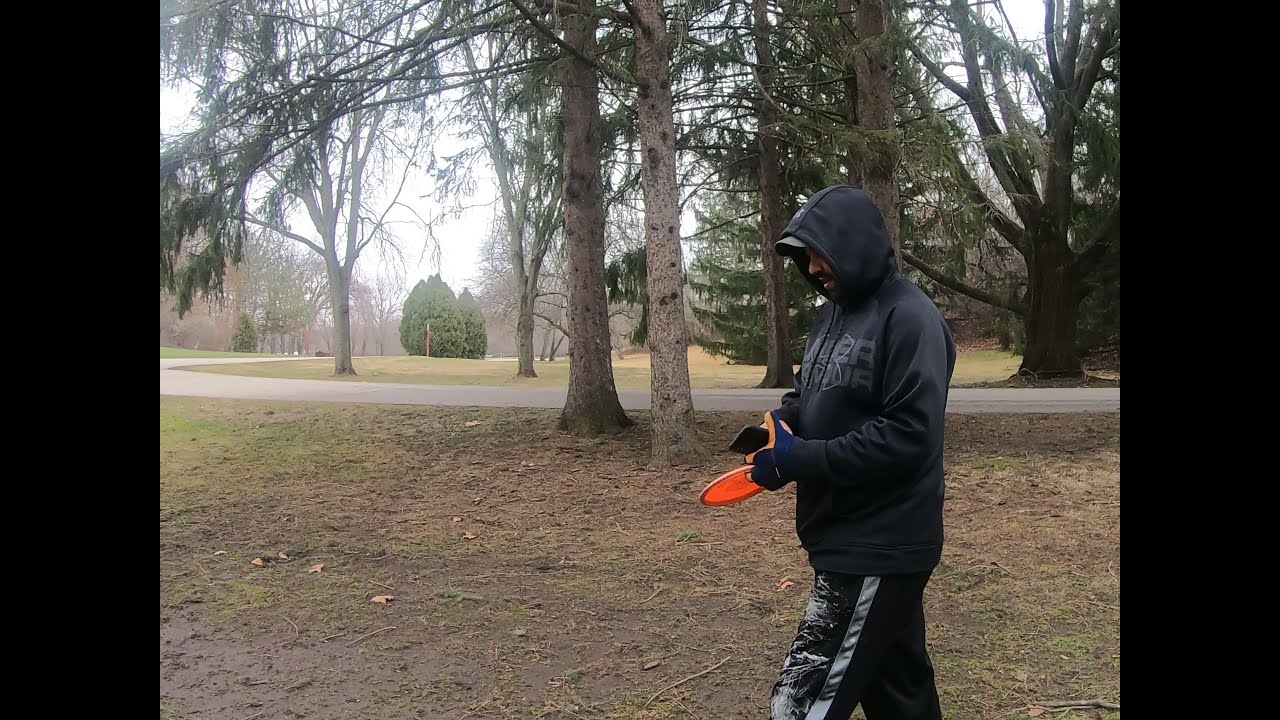In the park-like setting of the image, a man stands slightly off-center towards the right. The foreground is primarily a muddy expanse interspersed with patches of green grass. He is dressed in a black hoodie with its hood over his gray baseball cap, and black long pants featuring a gray stripe and pattern on the front. His hands are adorned with orange and blue gloves; one hand holds a smartphone while the other grips an orange Frisbee. The scene includes a curving road that bisects the image diagonally, with more grass and clusters of trees in the background. The road curves to the left and leads further into the distance. Above, the sky is a light, overcast gray, contributing to the muted and serene atmosphere of the park. The background is rich with tall, brown tree trunks and branches adorned with green leaves. Beyond the trees and road, there are more verdant areas and a field, enhancing the picturesque park setting.